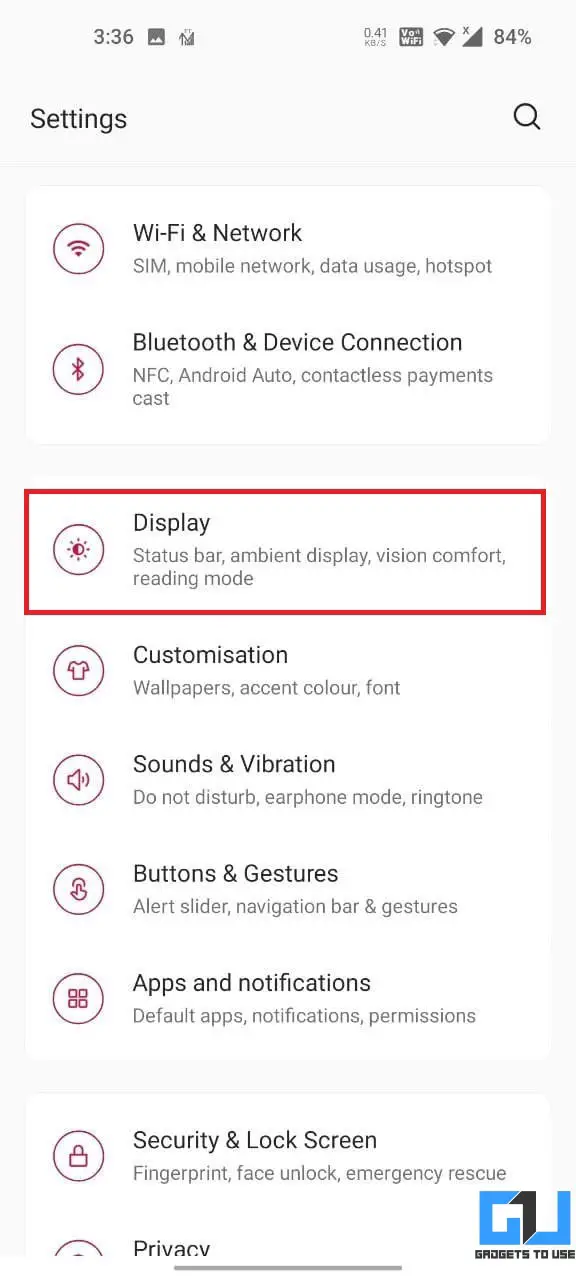The screenshot shows an Android mobile app interface, specifically the Settings menu, captured at 3:36 with various icons displayed along the top status bar. To the right of the time are two indistinct icons, likely for screenshots and uploads, followed by a reading of 0.41 kilobits per second, indicating data transfer activity. VO Wi-Fi and nearly full Wi-Fi and cellular signal bars suggest a strong connection, while the battery is at 84%.

The Settings page features a light gray and white background. On the left-hand side, "Settings" is prominently displayed with a search magnifying glass icon adjacent to it. Below, menu options include:
1. "Wi-Fi and Network" accompanied by a Wi-Fi icon.
2. "SIM, Mobile Network, Data Usage, and Hotspot."
3. "Bluetooth and Device Connection," which expands to include NFC, Android Auto, Contactless Payments, and Cast.

Further down, enclosed in a red rectangle, are options for:
- Display: Status Bar, Ambient Display, Vision Comfort, and Reading Mode.

Other visible settings options include:
- Customization
- Sounds and Vibration
- Buttons and Gestures
- Apps and Notifications
- Security and Lock Screen
- Privacy

The bottom right features a company insignia labeled "Gadgets to Use" and a "GU" logo in predominantly blue and black fonts.